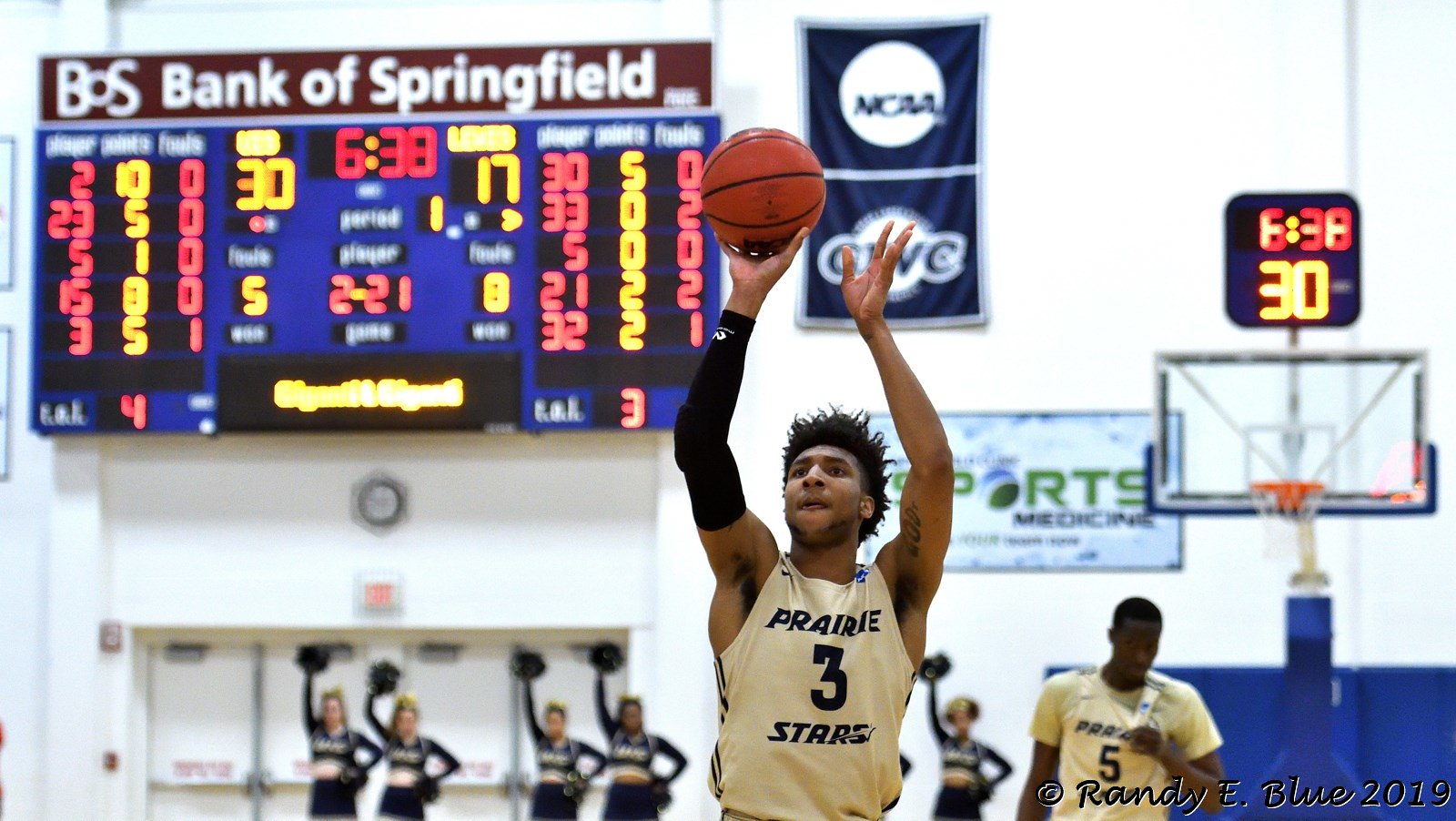The image captures an African American basketball player from the Prairie Stars team, poised to take a jump shot. He is clad in a cream-colored jersey with black text that reads "Prairie Stars" and features the large number three. His left arm is adorned with a black compression sleeve, and he holds an orange basketball, ready to shoot. In the background, a blue banner with the NCAA logo is visible, and a scoreboard sponsored by BOS Bank of Springfield shows a score of 30 to 17 with 6:38 remaining. Cheerleaders with pom-poms and another player, wearing a jersey with the number five, are also discernible in the background. The image is credited to Randy E. Blue, 2019.